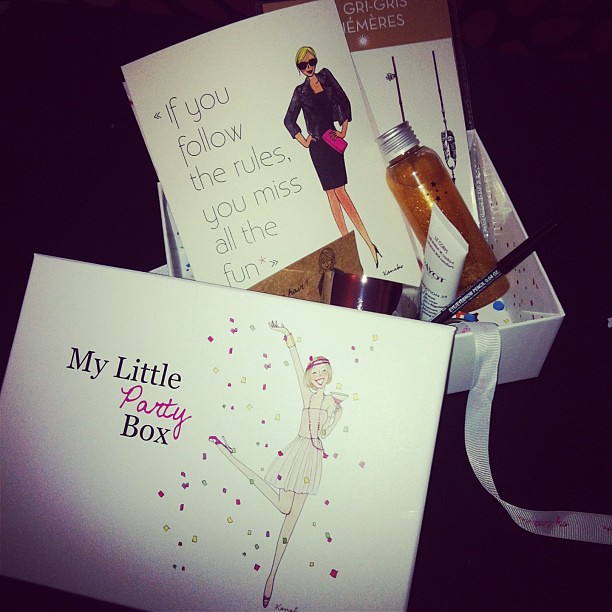The image features an open white box named "My Little Party Box," set against a black background. The box lid is propped up, revealing its cover illustration: a jubilant woman adorned in a 1920s flapper outfit, including a pink hat, long necklace, and short skirt. She stands on her toes with one leg playfully bent behind her, holding a martini glass filled with pink liquid. Confetti surrounds her, and she sports a big smile. The text on the lid reads "My Little Party Box," with "party" in pink script and "my little" in black regular font.

Inside the box, various cosmetic items are neatly arranged, including tubes and bottles likely containing beauty and health products for women. Among the contents, there is a hand cream tube, a small vial of liquid, a makeup brush, and possibly a ribbon that ties the products together. Additionally, there are pamphlets and papers, one of which prominently displays the phrase, "If you follow the rules, you miss all the fun." The entire setup suggests a playful, celebratory theme perfect for a woman's night of fun and beauty.